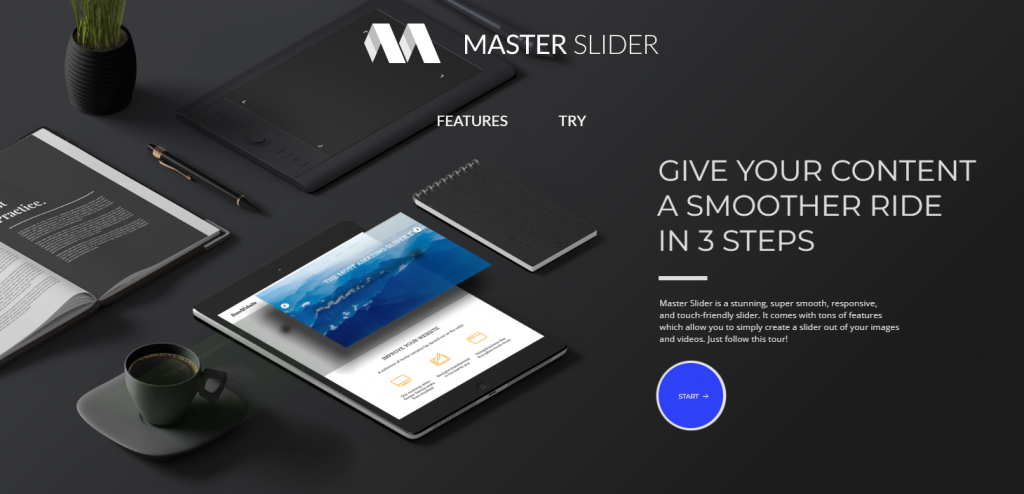The advertisement features a sleek black background, with the center top highlighting the brand name "Master Slider." The logo consists of a stylized letter "M" followed by "Master" in white, and "Slider" in a slightly darker light gray. To the right of this, in bold capital letters, is the tagline: "GIVE YOUR CONTENT A SMOOTHER RIDE IN THREE STEPS."

Beneath this, in smaller text, the advertisement describes: "Master Slider is a stunning, super smooth, responsive, and touch-friendly slider. It comes with tons of features which allow you to simply create a slider out of your images and videos. Just follow this tour."

At the bottom, there's a prominent blue circle with a white border. Inside the circle, in small text, is the word "Start" accompanied by an arrow pointing to the right.

This composition is superimposed on a background image depicting a black desk or table scattered with various items:

- An open book with small, out-of-focus text, making it difficult to read.
- A pen lying on the surface near the book.
- A gray cup of coffee resting on a matching gray holder.
- A turned-on tablet displaying images and text on its screen. Overlaid on the tablet is a blue, swirly image with the text "The Most Amazing Slider."
- A closed black notebook positioned next to the tablet.

Overall, this advertisement effectively combines stylish elements and detailed design to promote the sophisticated features of Master Slider.